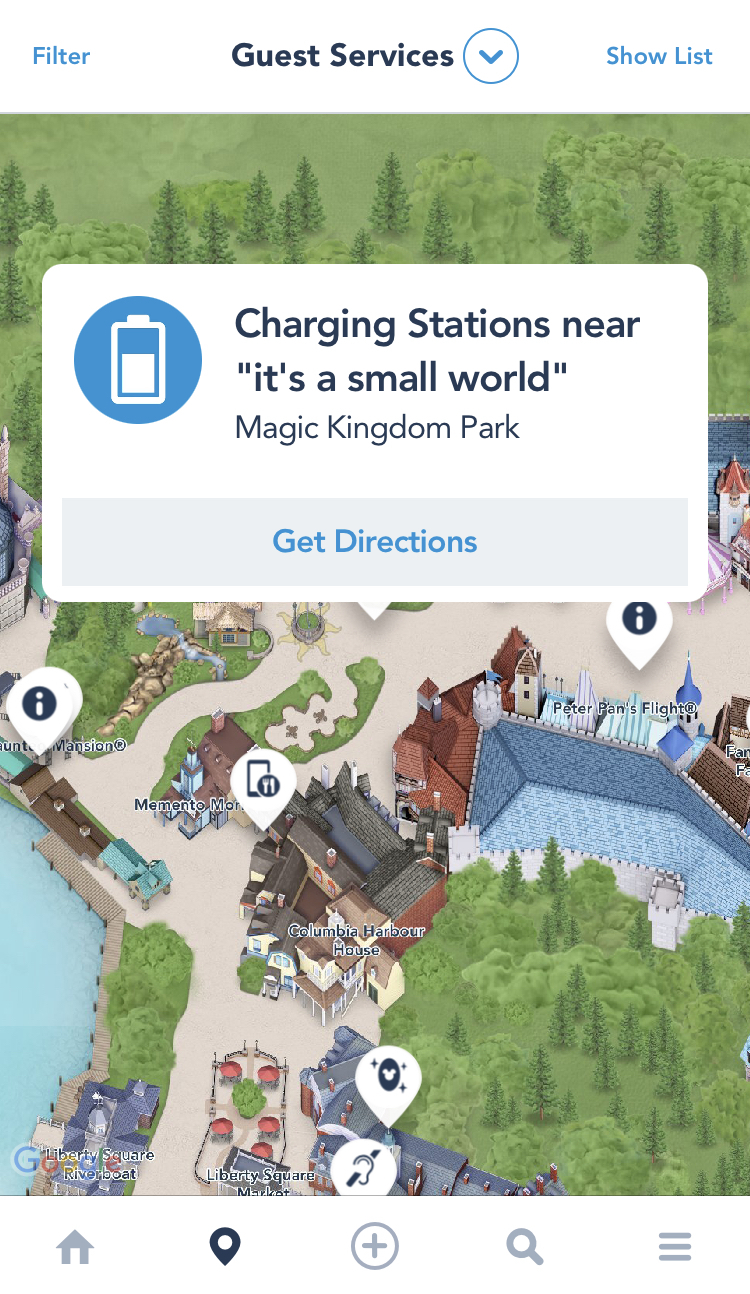This screenshot depicts an interactive map of Magic Kingdom Park from the Disneyland or Disney World mobile app, viewed on a cell phone. The map itself features a cartoonish, stylized overhead view of the park, rather than a traditional satellite image, capturing the whimsical essence of Disney. The interface is powered by Google, as indicated by the logo at the lower left corner of the screen. 

At the center of the map, a pop-up notification informs the user that a Charging Station is located near "It's a Small World" in Magic Kingdom Park, and offers a "Get Directions" button for navigational assistance. 

The header of the app includes a "Guest Services" drop-down menu, along with additional buttons such as "Show List" and "Filter." Various icons and pins are placed on the map to denote significant locations, including charging stations and information centers. Specific attractions marked on the map include Peter Pan's Flight, Memento Mori, Columbia Harbour House, and Liberty Square Market. Overall, the map is specifically designed to help visitors locate amenities and attractions within Magic Kingdom Park effectively.